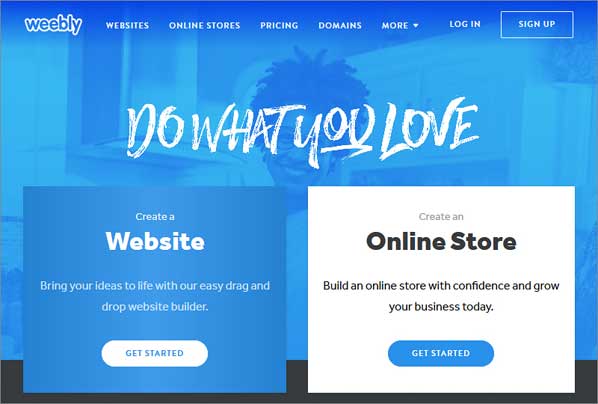The image depicts the homepage of the Weebly website. In the upper left-hand corner, the Weebly logo is prominently displayed. To the right of the logo, a navigation menu includes the options: "Website," "Online Stores," "Pricing," "Domains," and "More," with "More" featuring a dropdown arrow. Adjacent to the navigation menu are the "Login" and "Sign Up" buttons, the latter enclosed in a rectangle. 

Beneath the navigation bar, the tagline "Do What You Love" appears in a stylish, almost cursive font. The background features a smiling woman with glasses and short hair, which is fuller on top. She faces forward, adding a welcoming and positive vibe to the page.

Directly below the tagline, there are two call-to-action boxes side by side. The box on the left is blue and states "Create a Website," with "Website" bolded in white. It further encourages users with the phrase "Bring your ideas to life with our easy drag-and-drop website builder" followed by a "Get Started" button.

To the right, a white box invites users to "Create an Online Store," with "Online Store" bolded in black. It reassures potential users with the message, "Build an online store with confidence and grow your business today," and also features a blue "Get Started" button in an oval shape.